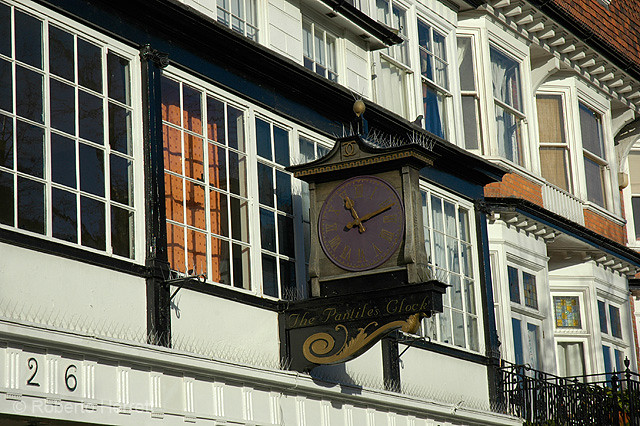This is a photograph of a historic British clock shop, distinguished by its largely white exterior and extensive windows adorned with small panes. Prominently featured is a hand-crafted, wooden clock sign extending from the side of the building. This sign has an intricate design reminiscent of pagoda architecture, and it is richly detailed with a purple clock face framed by gold Roman numerals and gold or bronze clock hands. The clock face is set against a gray, shiny black base trimmed in gold, which bears the name "The Pantiles Clock" in an old-fashioned script. Below the clock, a small golden flourish adds a decorative touch. The building itself, identified as number 26, boasts traditional architecture with multiple attached structures that include unique, outward-projecting window designs. The lower part of the building features dark brown trim, enhancing its classic aesthetic. This scene, evocative of European street views, captures the charm and character of this quaint establishment.